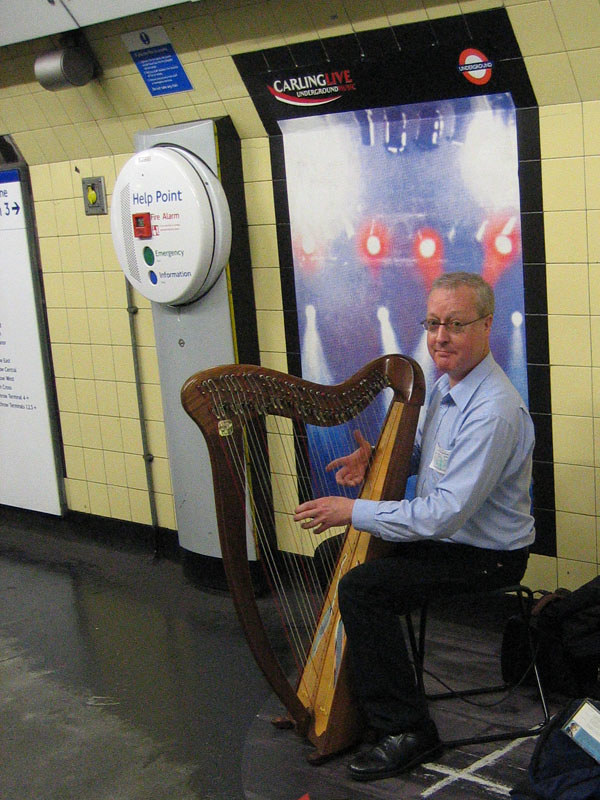In the image, a musician, dressed in a blue long-sleeve button-down shirt and black pants, is seated on a stool at what appears to be a subway platform or a bus station. The man, who is wearing glasses, is playing a small harp while looking directly at the camera. His surroundings include a hard concrete surface and a wall adorned with yellow tiles and various advertisements. Behind him to his right, a help point monitor is visible hanging from the wall. The lighting in the background suggests stage lights flashing, which adds an interesting dramatic effect to the scene. The overall setting is indoors, giving off a somewhat worn and utilitarian ambiance characterized by a mix of gray, black, brown, light blue, red, green, blue, and tan hues.